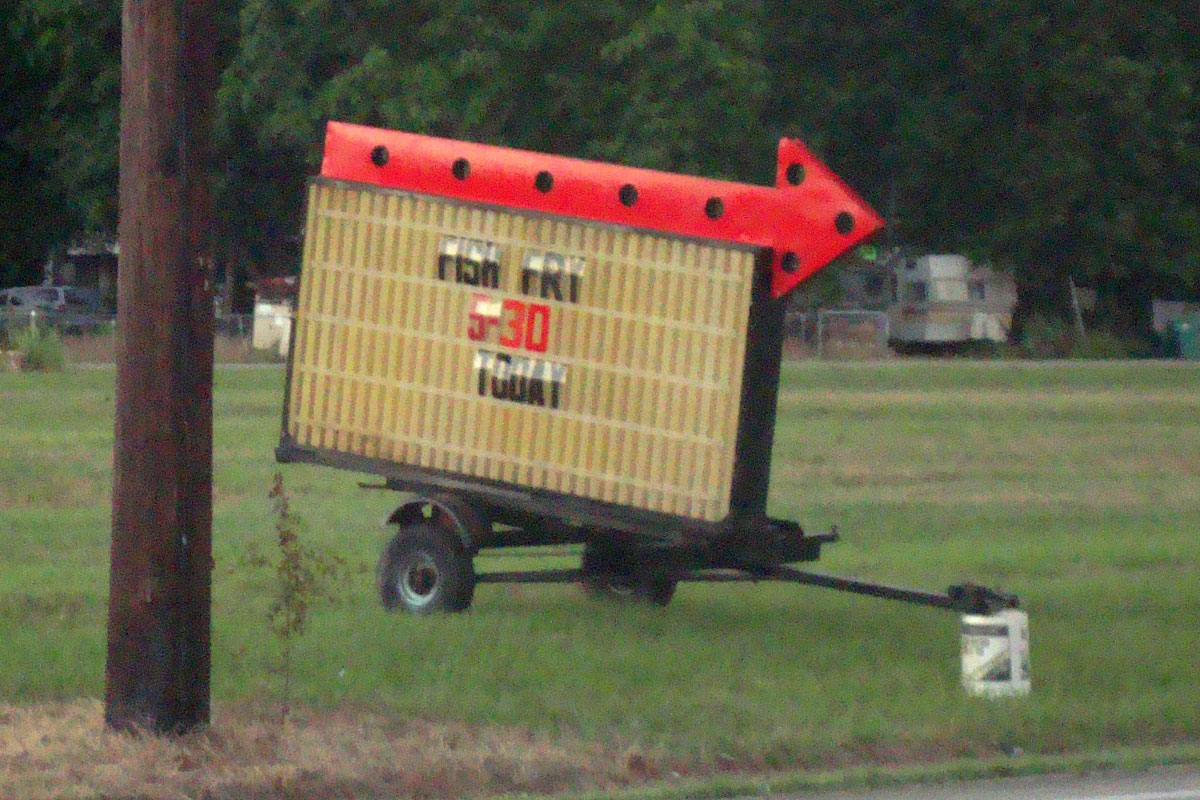A roadside photo captures a rustic scene featuring a marquee sign mounted on a black two-wheeled trailer parked on freshly cut, verdant grass. The trailer's front hitch is propped up on an inverted bucket. Nearby stands a tall telephone pole, partially visible from the ground up. The marquee, a light beige in color, prominently displays a large red arrow with black polka dots running across its top. The sign announces in black letters, "Fish Fry Today," with the time "5:30" highlighted in red numbers beneath.